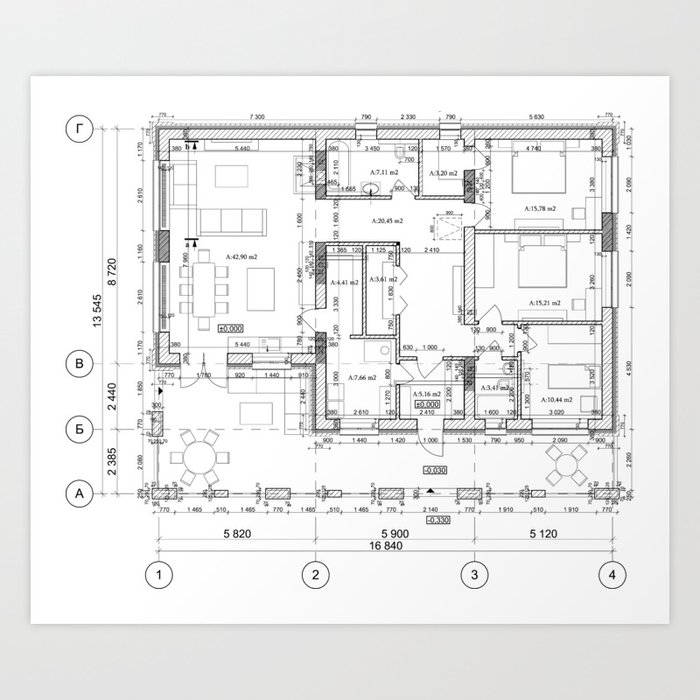This detailed black and white blueprint depicts a building's floor plan against a gray background block. The blueprint showcases various rooms with dimensions, entranceways, and precise measurements, making it seem like it’s for either a large house or another substantial structure. The plan appears to outline at least 12 rooms, including specific spaces such as a kitchen table area and chairs. The intricate design includes labeled numbers and letters, such as "A, B" on the left side and "1, 2, 3, 4" on the bottom, each enclosed in small circles. The blueprint, created using black ink or pencil on a white backdrop, reflects detailed architectural planning for construction purposes, featuring measurements, degrees, and potential shadings for different sections.